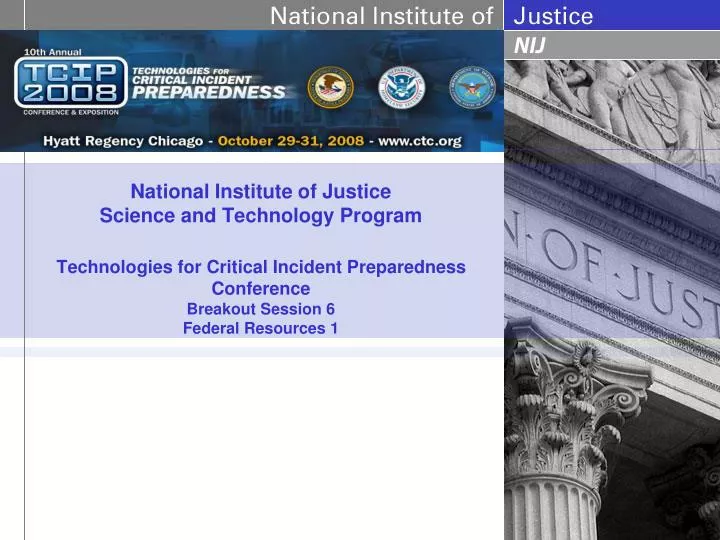The image features several distinct elements organized in a structured layout. In the top left corner, there is a vertical white line that extends down about five percent of the image's height. Below this line, a transparent blue rectangle overlays the background, partially revealing an image of what appears to be a police car.

Above the blue rectangle, a right-aligned gray rectangle contains the text "National Institute of" in white. Within the blue rectangle are three seals arranged horizontally: from left to right, the first seal is yellow, the second is white, and the third is blue. The majority of the text within this rectangle is white, with the exception of the dates "October 29th - 31st, 2008," which are highlighted in yellow.

Below this section, there is a purplish-gray rectangle featuring purple text that gradually decreases in font size toward the bottom. To the left of this text block, a gray vertical line runs the full length of the image.

In the top right corner, a purple rectangle contains the word "Justice" in white text. Below this rectangle, a white horizontal line separates it from another gray rectangle that features the abbreviation "N-I-J" in white text, followed by another white horizontal line. Beneath this, there is a depiction of a building, likely constructed of marble, adding a significant visual element to the design.